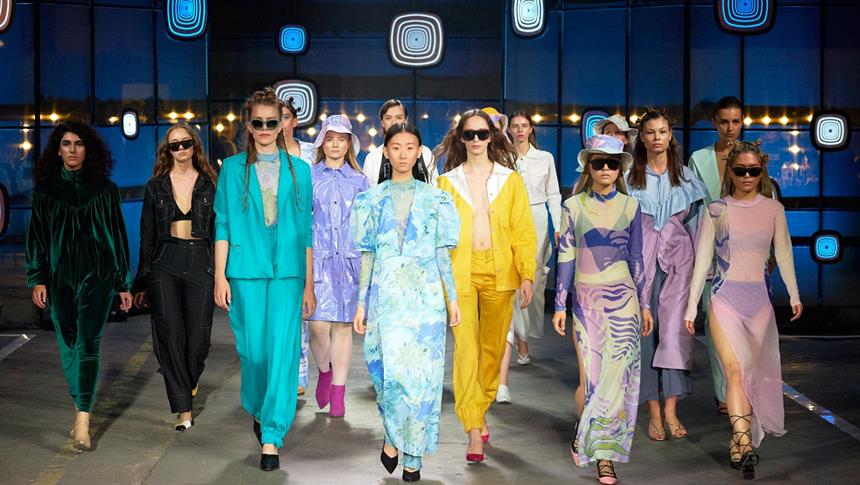In this vibrant photograph, a group of twelve women is captured walking towards the camera on a gray walkway, likely a runway. The women, who are of diverse races, are all dressed in various colorful and stylish outfits, primarily dresses, with one woman donning a turquoise suit and another in a light blue floral dress. The woman at the center, an Asian model, stands out in a dress paired with pants beneath it. Many of the women sport sunglasses, while a few wear large rimmed hats. Their expressions are serious, reminiscent of supermodels. The backdrop features striking blue walls adorned with glowing logos comprised of squares in shades of light and bright blue, adding to the dynamic and vibrant atmosphere. The background also includes colors like gold and white, contributing to the overall colorful and diverse visual presentation.